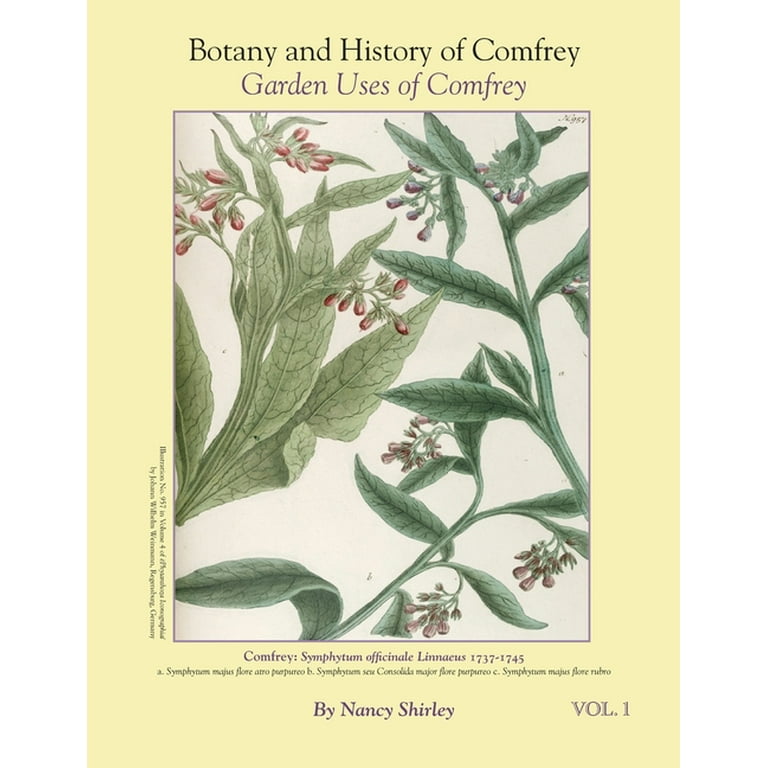The image features a cover that seems to be from either a book or a magazine, framed with a pale yellow or tannish background. The top of the cover displays, in dark blue lettering, the titles "Botany and History of Comfrey" and "Garden Uses of Comfrey." Below the titles, there is a detailed drawing of comfrey, exhibiting green leaves with thick, long stems, and adorned with small, oval buds in shades of red and purple. At the bottom of the image, the text reads "Comfrey Symphytum Officinale Linnaeus, 1737-1745," followed by "By Nancy Shirley, Volume 1." There is also a line of small, black text beneath this information. The overall design gives the impression of an old, possibly historical document or article cover dedicated to the botany and uses of comfrey.